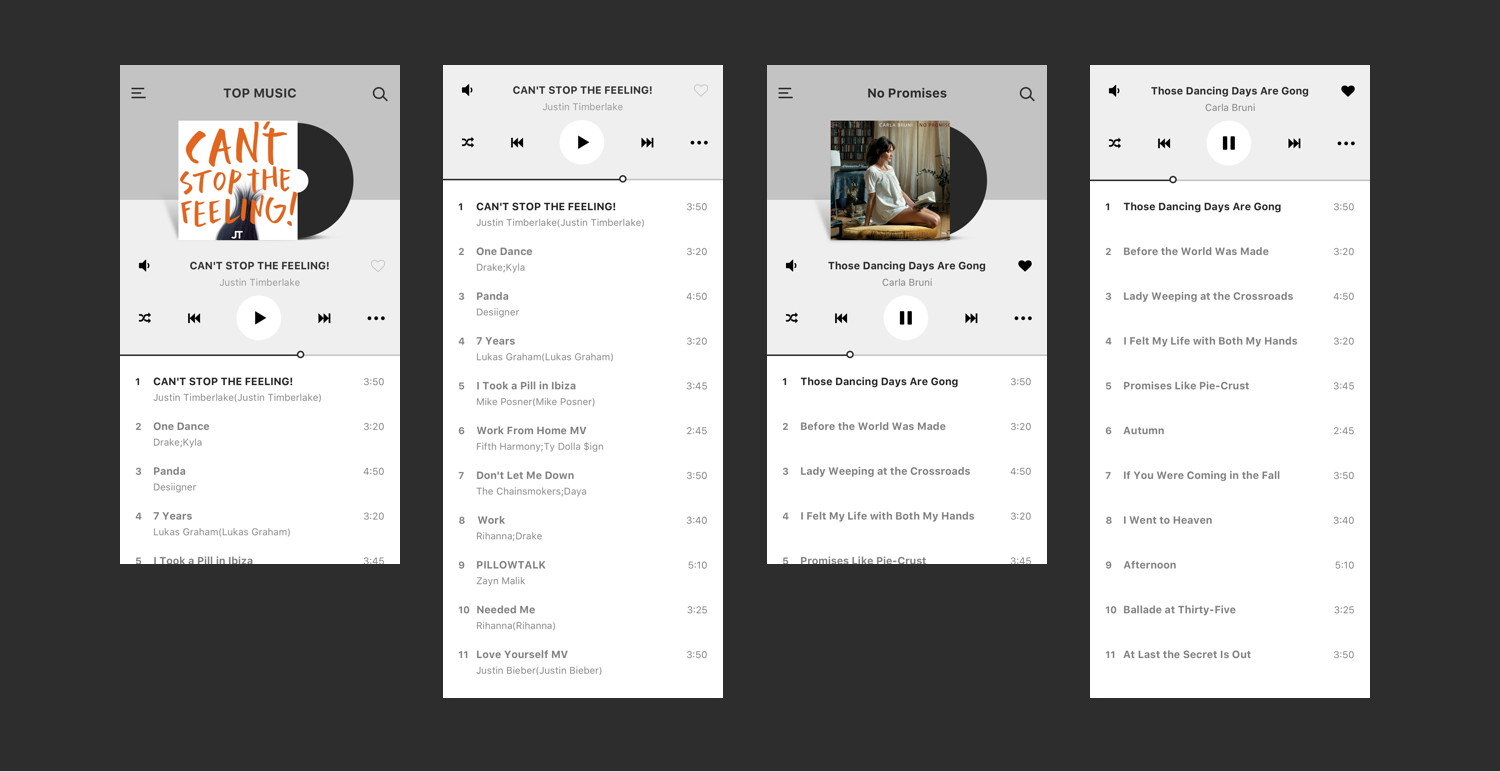The image consists of four different screenshots of a phone within a black rectangular background, each showcasing distinct music ranking lists and album covers.

1. The first screenshot features a top music chart titled "Top Music." The number one song is "Can't Stop the Feeling" by Justin Timberlake. Following it are "One Dance," "Panda," "Two Years," and "I Took a Pill in Ibiza." Notably, "Can't Stop the Feeling" appears prominently at the top of this chart without an accompanying icon, containing similar metadata.

2. In the second screenshot, the chart appears to be a continuation or another version of popular tracks. It includes songs like "Work From Home," "Don't Let Me Down," and others, extending to make a top 11 list, though some text is difficult to read.

3. The third screenshot highlights an album titled "No Promises," with the subtitle "Those Dancing Boys Are Going." Below the album information, there are several other music choices, though they are not specified in detail.

4. The fourth screenshot also focuses on the album "Those Dancing Boys Are Going," indicating it as being ranked number one. This ranking appears before another piece titled "Before The World Was Made," followed by additional unspecified entries.

Overall, the four screenshots collectively represent various music charts and album rankings on possibly the same phone, displaying popular songs and albums in different settings.